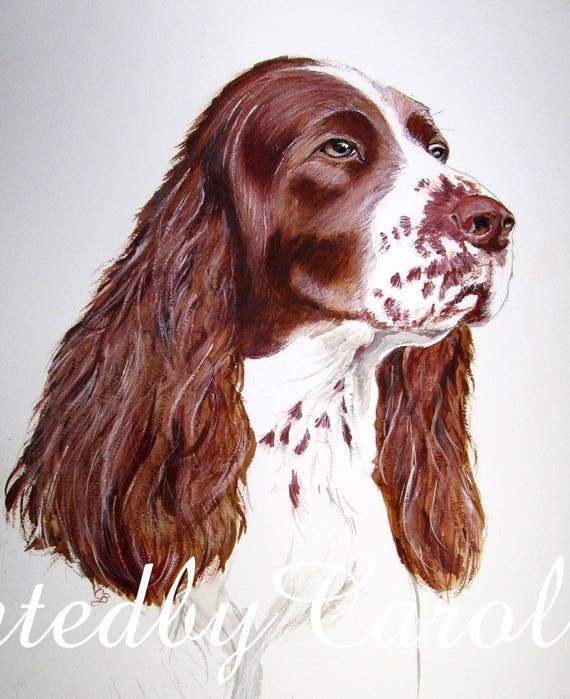This image presents a side view of a dog that resembles a Cocker Spaniel, though some might think it looks like a Beagle. The dog is primarily white with distinctive brown markings. Around its eye and ears, it has rich brown fur, and its long, wavy ears feature curly hair. The dog's nose is a reddish-brown color, distinct from a typical black nose. Brown speckles adorn its white muzzle and under its chin. Its eyes are a light brown, with a white strip of fur running between them down the center of its face. The background of the image is a solid white color, highlighting the dog's features. The image only shows the dog from the top of its head down to just below the chest area, including part of the shoulder. At the bottom of the image, there is partially visible white text, with the words "Carol" and "T-E-D-B-Y" decipherable.